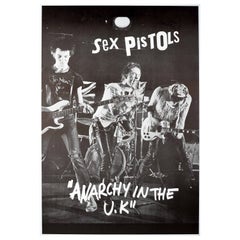This black and white image captures the iconic punk rock band Sex Pistols during a performance in the 1970s. The photo prominently features Johnny Rotten, the lead singer, gripping a microphone, and Sid Vicious, the bassist, sporting a black shirt, black hair, and jeans with a hole in the knee area. The stage setup includes a drum kit in the background, adding to the raw energy of the scene. The composition shows three band members: one on the left in a black shirt holding a guitar with a black and white body, Johnny Rotten in the center wearing a white shirt and black pants, and another member on the far left in a white shirt, hunched over a guitar. Above them, in bold white uppercase letters, it reads "SEX PISTOLS," with slightly larger fonts for the S, P, T, and O. Below this, the text "Anarchy in the UK" also appears in white. The image may be a poster or a card, indicated by a small hole at the top center, suggesting it could be clipped or hung. The band members are positioned against a gritty backdrop, reflecting the rebellious spirit of their music and the era.